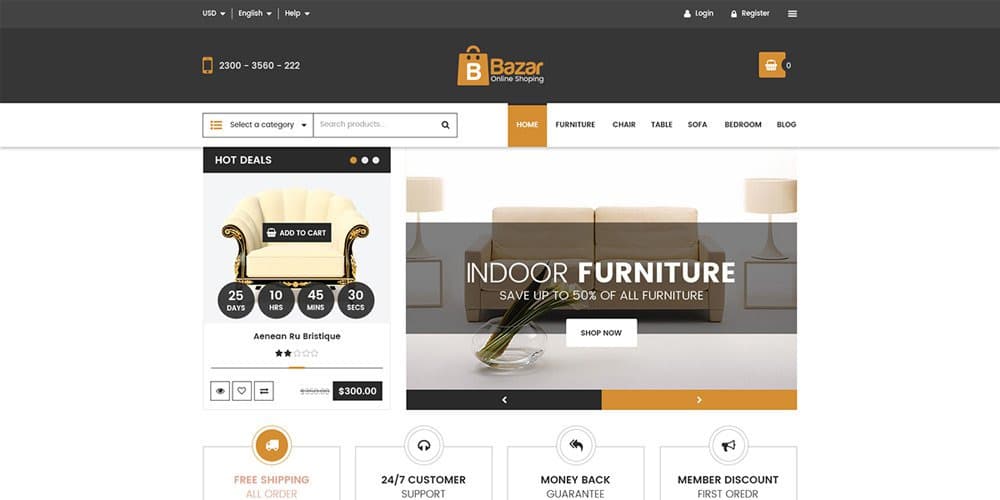The image displays a web page with a distinct dark gray header at the top. Within this header, it reads 'USD English Help Login Register.' Below the header is a larger black section featuring a cell phone icon accompanied by the number '2300-3560-222.' Centrally located, there is an orange shopping bag with a white 'B' in its center, next to the text 'Bazaar Online Shopping.' To the right of this area is an icon of a shopping basket inside an orange square.

Beneath this, a search bar allows users to 'Select a Category' and type their query. Below the search bar, a navigation menu includes links labeled 'Home,' 'Furniture,' 'Chair,' 'Table,' 'Sofa,' 'Bedroom,' and 'Blog.'

Further down, a black box labeled 'Hot Deal' is prominently featured. Below this box, an image of a chair is displayed, with a countdown timer in black circles indicating '25 Days,' '10 Hours,' '45 Minutes,' and '30 Seconds' remaining for the deal.